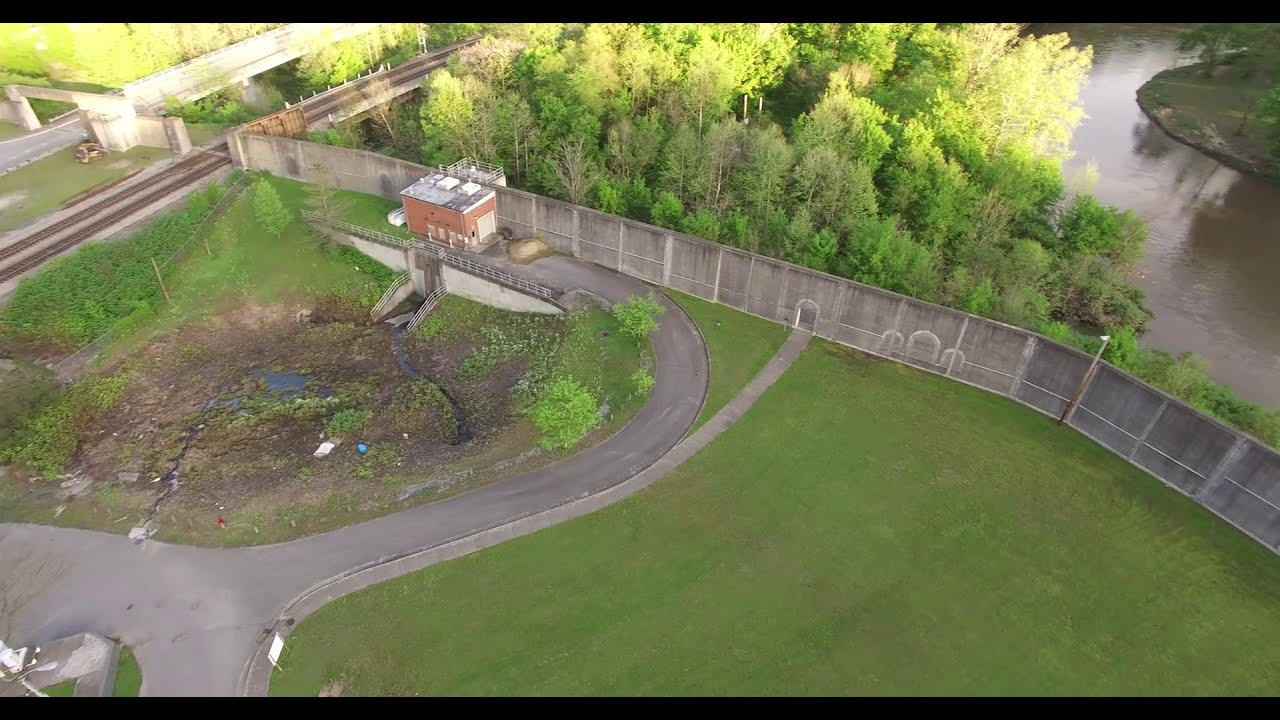The image is an aerial view, likely captured by a drone, depicting a diverse landscape. In the foreground, there is a well-maintained green lawn that is bordered by a fence running diagonally from the upper left-hand corner to the lower right-hand corner. This mostly wooden fence separates the lawn from trees in the background. To the upper right corner of the image, there is a body of water, possibly a river, reflecting sunlight and the surrounding trees. 

In the top left corner, a railway track cuts diagonally across the scene. Adjacent to this track, there is a small brick building with a flat roof, which appears to be either a power station or restroom, next to an outlet that might be part of a water treatment facility. Below this building, there is a mostly dry, muddy patch that looks like it was designed to catch water but currently contains only traces of moisture.

To the left of the image center, a dried-up pond or water body is visible, characterized by its circular, muddy outline. Surrounding this area, there is a mix of walkways and cement fencing extending from the bottom right to the center left. Beyond the fence, the landscape is densely populated with various trees, creating a vivid background of light and dark green hues.